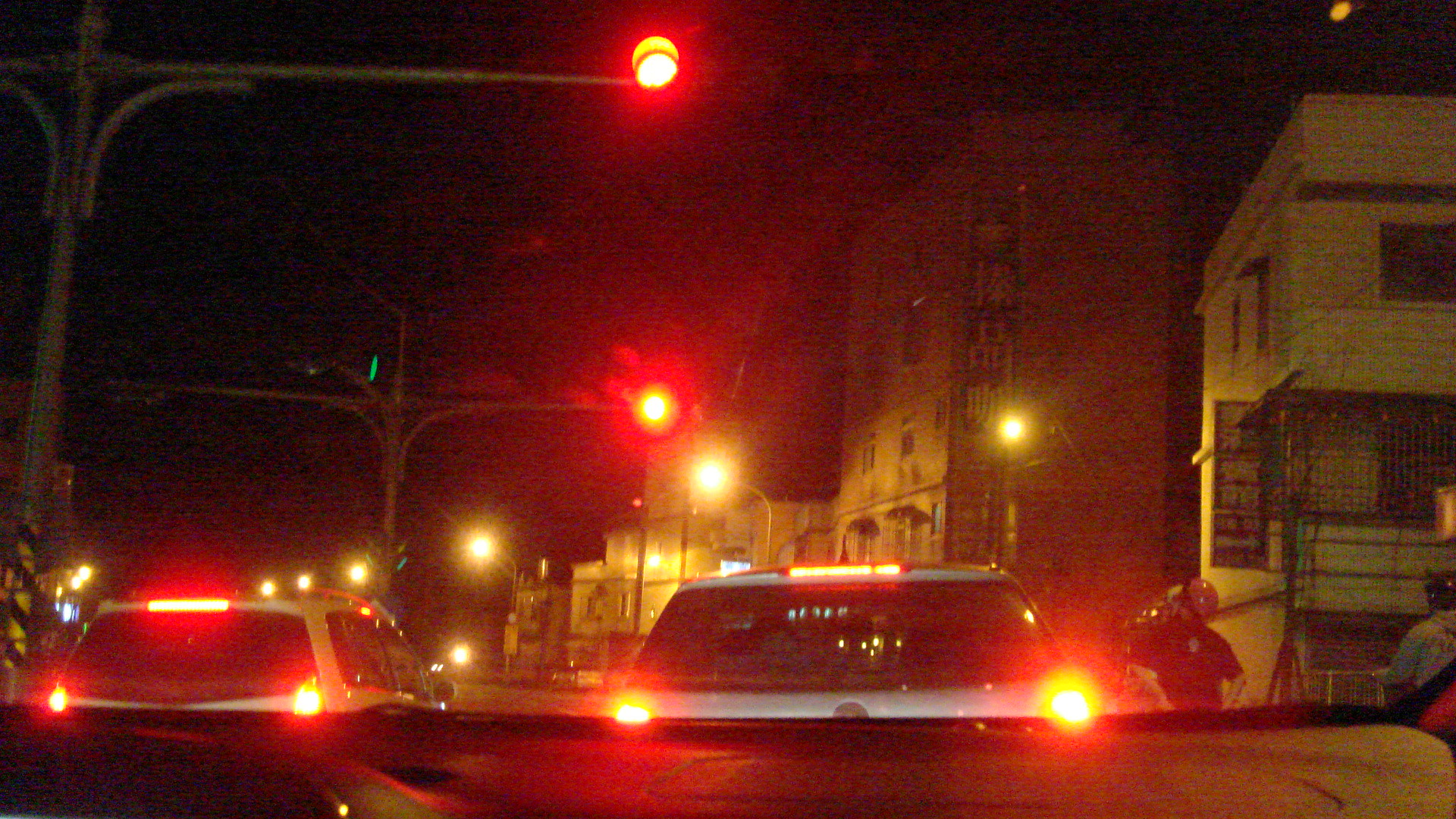A captivating nighttime urban scene, captured from inside a passenger vehicle. Along the bottom edge, a portion of the car's dashboard subtly frames the image. Directly ahead, a light-colored small passenger vehicle idles at a red light, its brake lights glowing vividly. To the left, in another lane, a yellow car also stands still, brake lights equally illuminated. High above, the red traffic signal casts a warm glow on the surroundings. On the right-hand side of the street, a couple of helmeted individuals stand, perhaps waiting to cross or for transportation. In the distance, the soft illumination from streetlights reveals a busy business district. Numerous buildings, adorned with banners of text in Asian characters, hint at a bustling commercial area. The interplay of light and shadow creates a dynamic and immersive nocturnal cityscape.